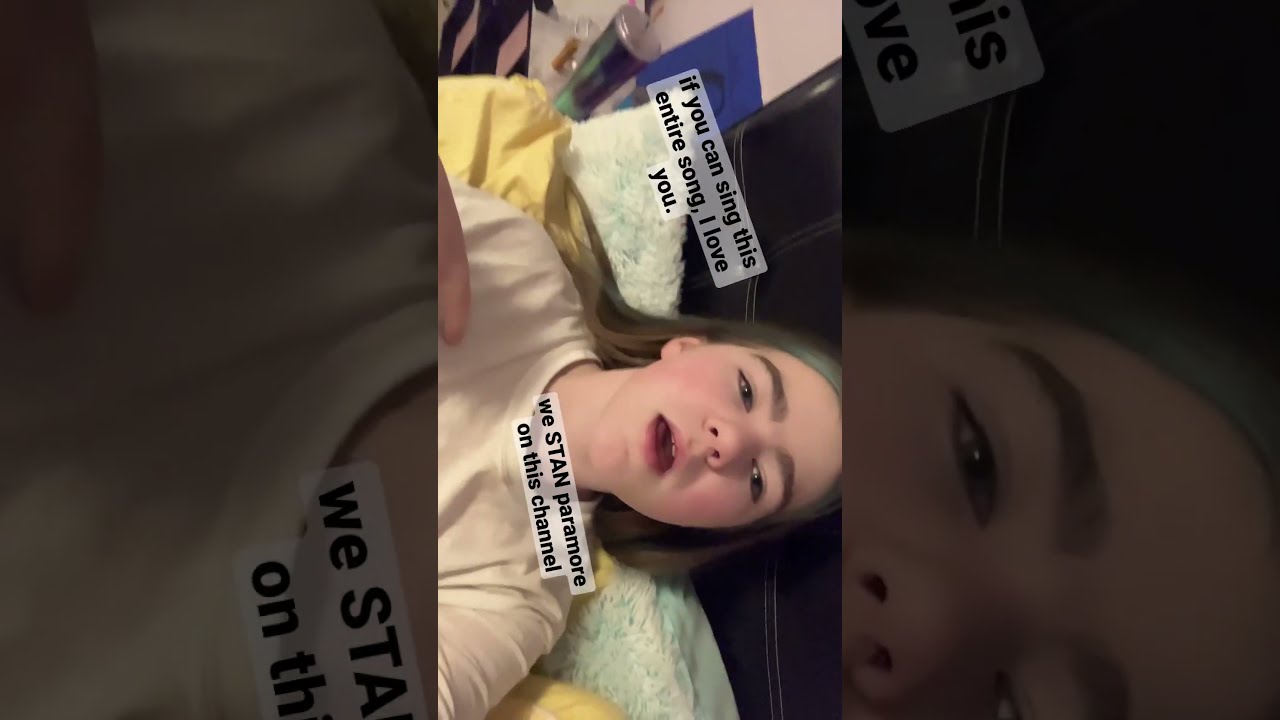The image shows a young woman reclining sideways on her bed, which appears rotated clockwise. Her mouth is gaping open, revealing thick brown eyebrows and pink lips. She has long hair that starts as a teal color in the front and transitions to her natural brown towards the ends. She is wearing a beige t-shirt.

Her bed features a black headboard, a cozy teal-colored Sherpa pillow, and a yellow comforter. A blue sheet peeks out at the left top side of the bed. To the right, which is the top of the rotated image, there is a small table with a cup on it. 

The scene includes digitally overlaid white text captions that read, "If you can sing this entire song, I love you" and "We stan Paramore on this channel." These captions are in black and white and are part of a large, greyed-out border that surrounds a narrower middle strip containing the main part of the image. The border itself is filled with an enlarged, darkened zoom of the same central image.